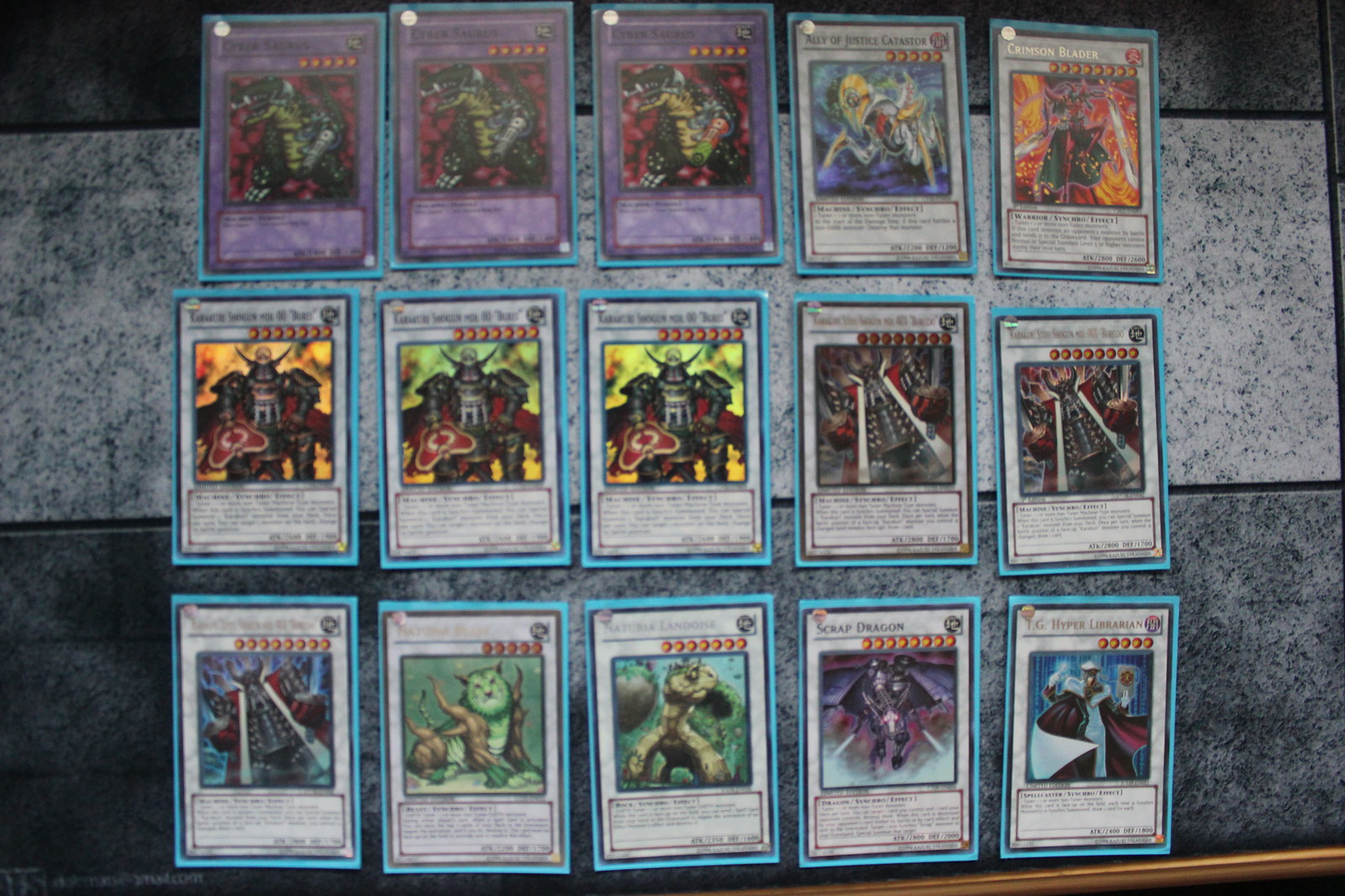The image depicts a collection of 15 trading cards, neatly arranged in a 3x5 grid on either a marble table or floor, divided by gray tiles at the top and bottom. Each card features digital images depicting medieval fantasy characters, reminiscent of games like Magic: The Gathering. In the top left corner, three cards share the same purple background and character. To the right, cards transition through various background colors - blue, green, orange, and lime green. The middle row mirrors the variety, with repetitive character cards set against orange, green, and lime green backgrounds. The cards below are distinct from the top and middle rows. To the lower right, a faint gold trim appears, framing the bottom of the layout. Despite the low resolution rendering text unreadable, one visible label in the top right reads "Crimson Bladder." The overall setup suggests a well-organized card collection with a diverse array of character depictions.